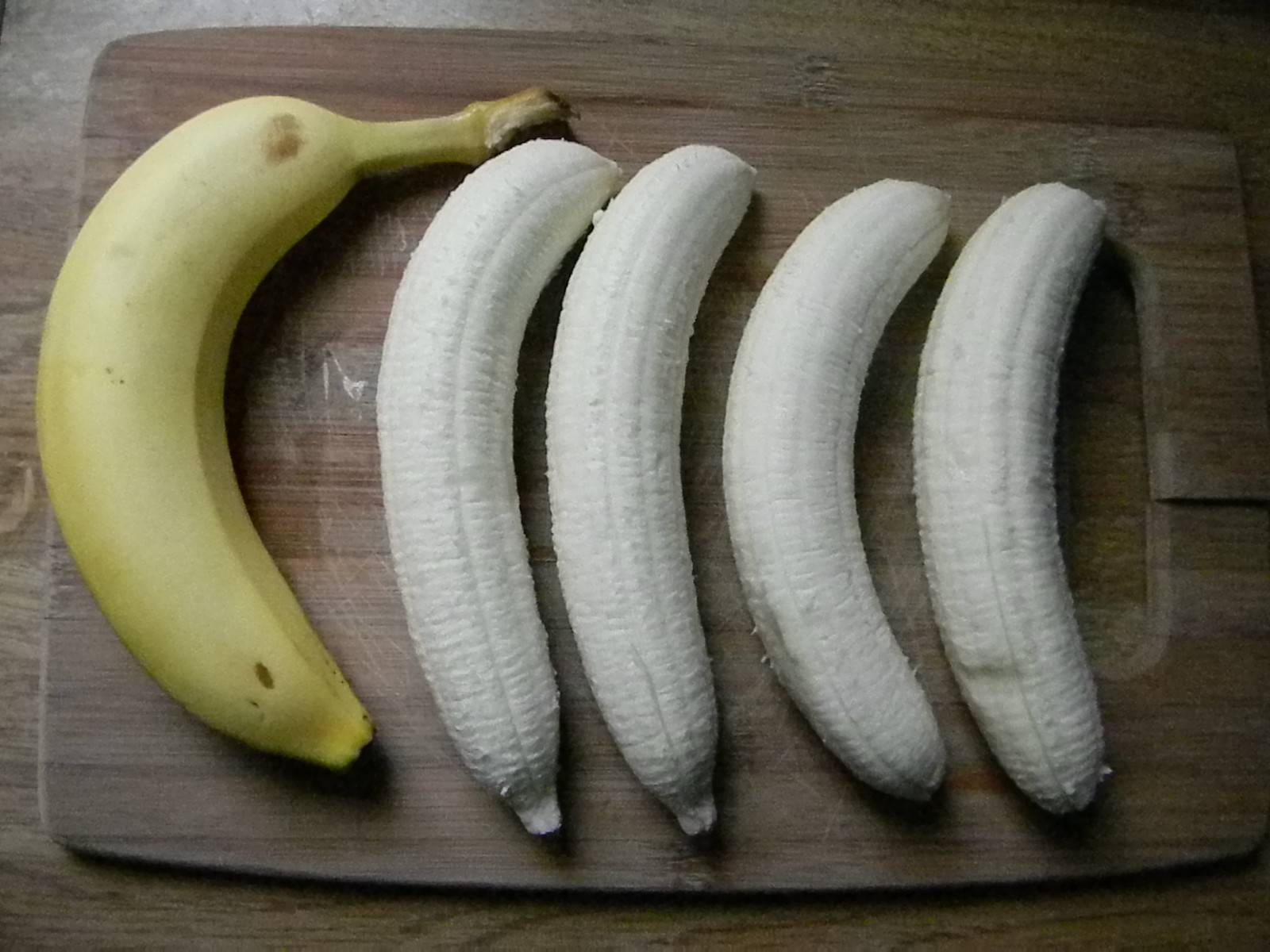In this image, a light wooden cutting board sits atop a similarly colored wooden table, creating a seamless blend of light wood grain textures. On the left side of the cutting board lies a perfectly ripe, slightly curved banana still in its peel, forming a 'C' shape. To its right, four unpeeled bananas are arranged in the same crescent moon configuration, each nestled closely to the next. The fourth unpeeled banana slightly overlaps the handle cut-out in the cutting board. The ripe banana showcases a flawless yellow peel with only a few minor brown spots, indicating its peak ripeness. This careful arrangement on the light wood background creates a harmonious and inviting composition.